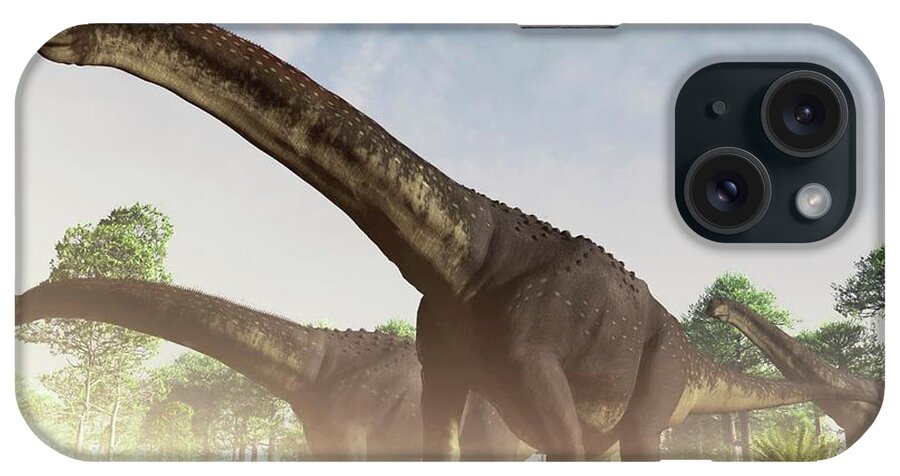The image captures a horizontal, rectangular cell phone case featuring an illustration of dark brown or gray brontosauruses set against a light blue sky with wispy white clouds. The scene includes a line of green trees along the bottom, adding depth to the background. In the upper right corner of the case, there is an opening for the cell phone camera lenses, with two lenses visible. The dinosaurs are positioned with one in the foreground, albeit with its head cut off; another to the right, showing just its long neck; and a third in the bottom left, partially obscured by the foreground dinosaur. The camera orientation on the case is horizontal, and no text is present in the image. The overall style denotes a product image, showcasing the phone case's design and functional elements.